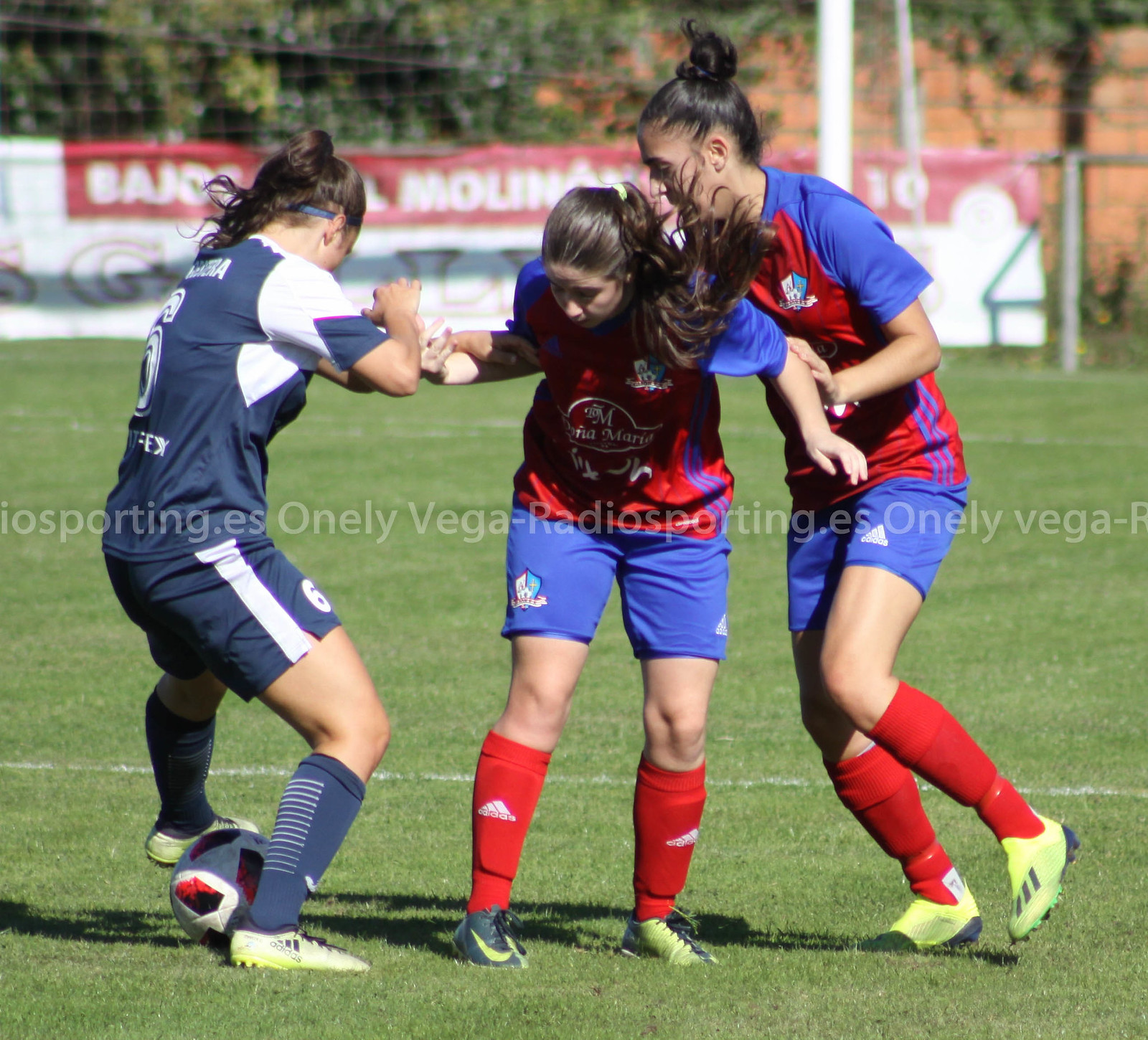This square photograph captures a vibrant moment during a girls' soccer game, framed within a sunlit, park-like setting. At the center of the action are three players: two on the right in red and blue uniforms with red socks, and one on the left in a blue and white striped uniform with blue or gray socks. The player in blue and white controls a white soccer ball with black and red accents, while the two opposing players try to intercept it. The scene takes place on a well-manicured green field, bordered by barriers and fences adorned with banners. In the distance, trees enhance the natural, open atmosphere. Superimposed across the center of the photograph is the translucent text "OnaleVegaRadioSporting.es," repeated prominently. Despite the intensity of the game, there are no stands visible, suggesting this is an amateur or school-level match.